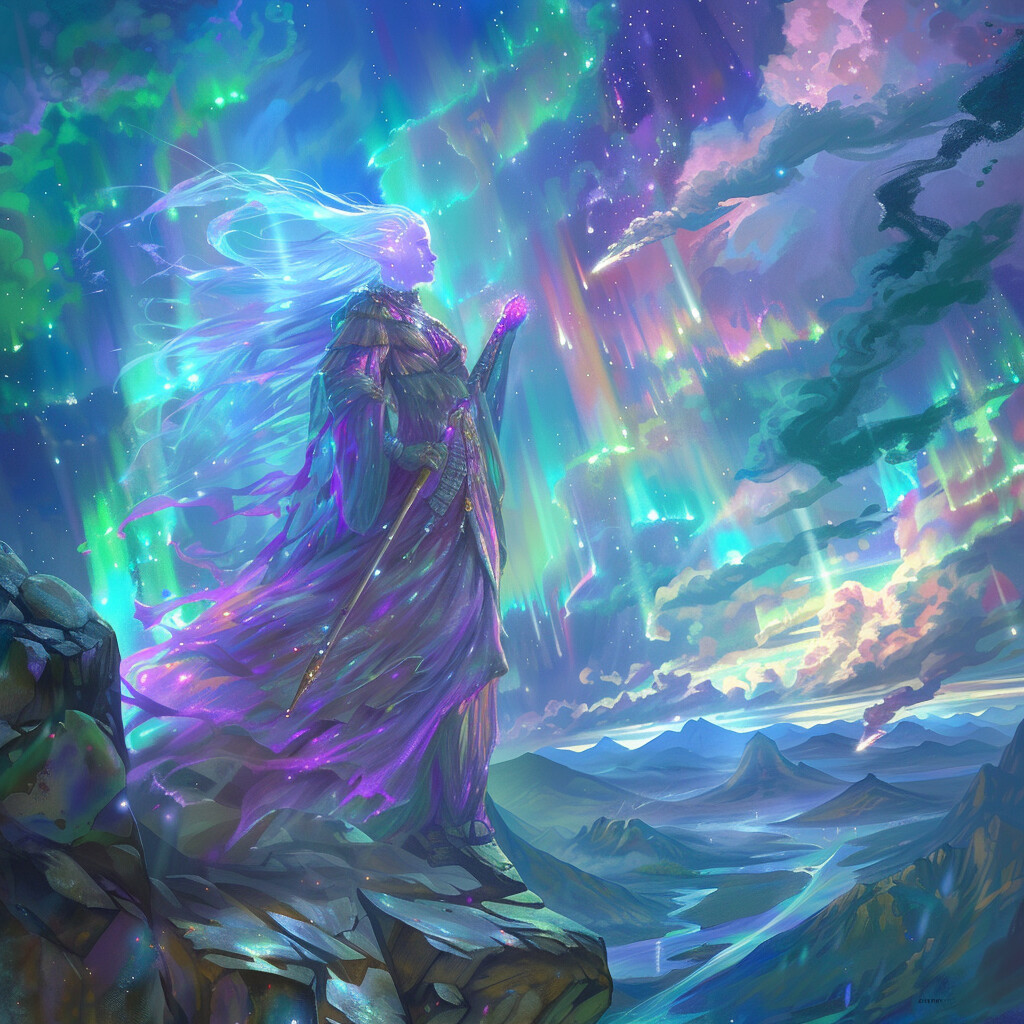This fantastical digital rendering depicts a mystical figure from a side point of view, gazing towards the right. Her long, flowy hair, a striking blend of blue and white, streams gracefully behind her. She's clad in a flowing garment that cascades around her form, mingling hues of green and purple, giving her an ethereal presence. The garment's long sleeves and hem add to its flowing nature, perfectly complementing her hair.

The woman stands poised on a rocky cliff, beneath which a diverse array of mountains can be seen, their colors ranging from blue to purple-gray. The sky above is alive with vibrant colors, a cosmic blend of blues, purples, and greens that suggest an otherworldly atmosphere. Bright beams of multicolored light pierce through the sky, mingling with peculiar cloud formations, stars, and glittering structures that enhance the surreal quality of the scene. In her hands, she grasps a staff or spear shaded in grays and purples, adding to her enigmatic aura. The overall scene exudes a sense of otherworldliness, making it seem as though she stands on an alien planet, with a thin river visible in the distant landscape.